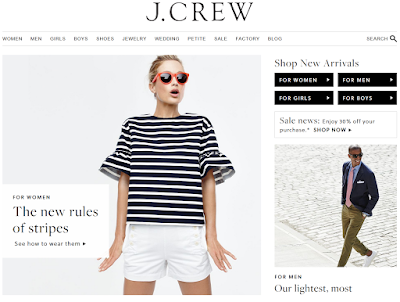This screenshot captures the homepage of the J.Crew clothing website. At the top, the company name "J.Crew" is prominently displayed in bold black letters. Below the header, a navigation bar features multiple tabs offering sections for Women, Men, Girls, Boys, Shoes, Jewelry, Wedding, Petite, Sale, Factory, and Blog.

On the top right corner, there's a search bar for finding specific clothing items. Directly beneath the navigation bar, there's a banner with clickable black tabs labeled "Shop New Arrivals" for Women, Men, Girls, and Boys, positioned in a grid format with Women and Men on the top row, and Girls and Boys on the bottom row.

Further down, a promotional section labeled "Sale News" advertises a 30% discount on purchases with a "Shop Now" link for easy access. 

Prominently featured in the center is an image of a bald man wearing black sunglasses, a blue dress shirt, a black vest, a red tie, brown pants, and white shoes. The text below the image reads "For Men, Our Lightest Most," with the rest of the sentence obscured.

On the left side of the screen, there's a large image of a woman wearing a black and white striped shirt, reminiscent of a mime or jail costume.